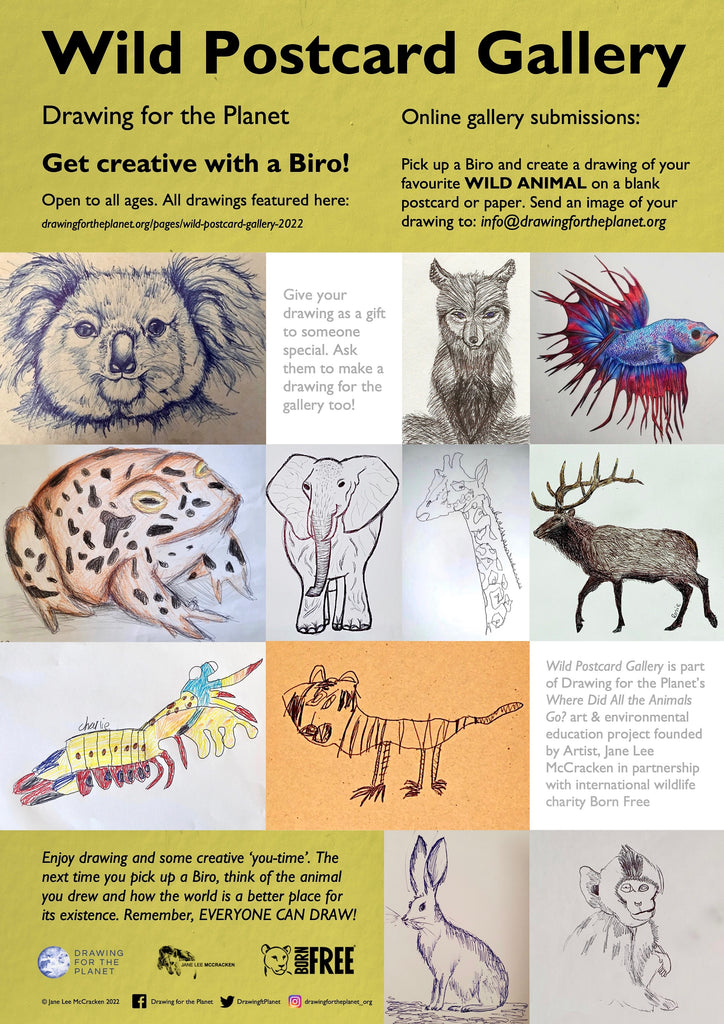The photograph showcases a vibrant promotional poster titled "Wild Postcard Gallery - Drawing for the Planet." The top of the poster features a heading that reads, "Get Creative with a Burrow, Open to All Ages, All Drawings Featured Here." This promotional event invites participants of all ages to submit their animal drawings. The poster displays a delightful array of artworks, depicting various animals such as a koala, a wolf, a fish, a frog, an elephant, a moose, a rabbit, and a monkey. The drawings exhibit a range of skill levels, from whimsical child-like renditions to highly detailed illustrations by professional artists. The overall theme emphasizes creativity and encourages artistic expression while celebrating the animal kingdom.